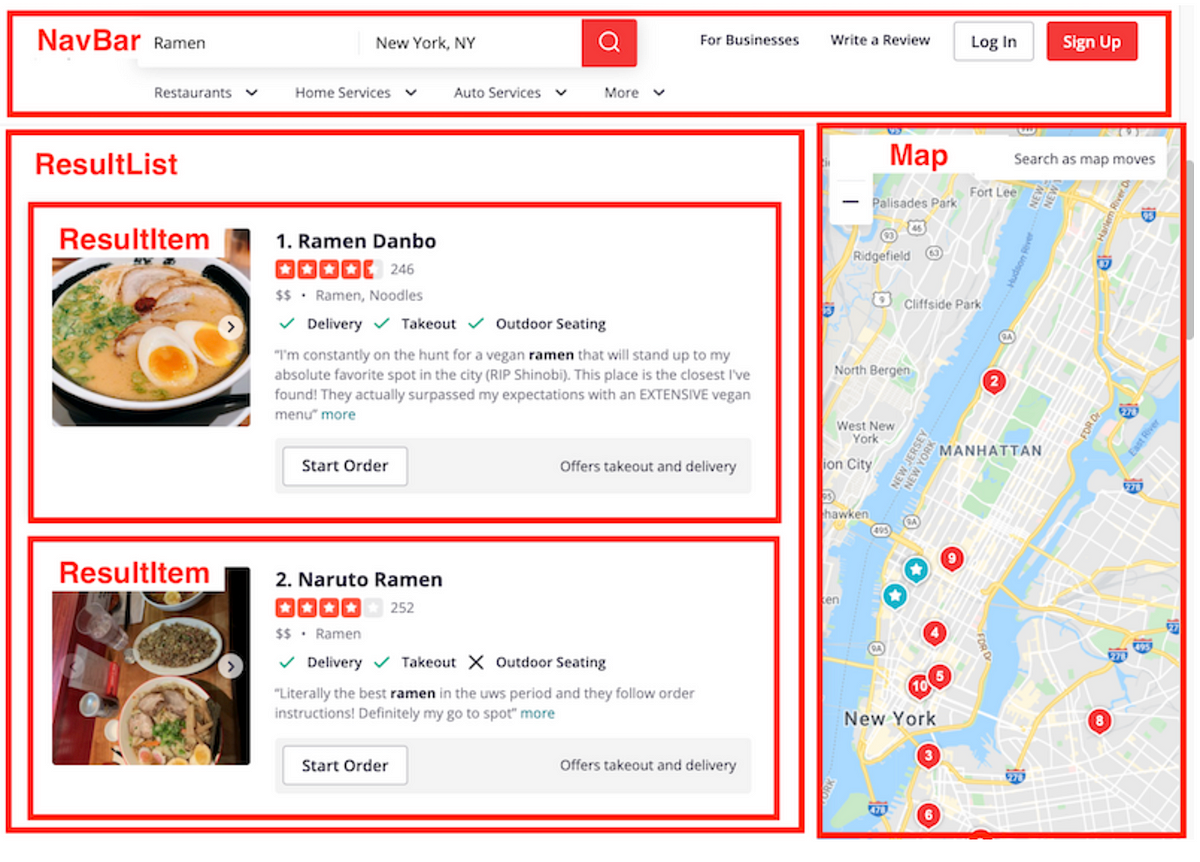This image is a screenshot of a restaurant listing page from what appears to be a review or food delivery website. The page is organized into several sections and branded with a navigation bar, allowing users to search for specific food items such as ramen and locations in New York City.

At the top, a search bar enables users to input queries for food items or services. Menu options are available for browsing categories like restaurants, home services, and auto services, among others. There are also links for businesses to list themselves, for users to write reviews, and for log-in and sign-up actions.

The main section lists restaurants, starting with "Ramen Danbo," which boasts a rating of 4.5 stars from 246 reviews. It is categorized under ramen and noodles and offers delivery, takeout, and outdoor seating. A brief review snippet praises their vegan ramen, and there is an option to start an order directly from this page.

Another featured restaurant is "Naruto Naruto Naruto," which has a 4-star rating from 252 reviews. Like the previous listing, it offers ramen, takeout, delivery, and outdoor seating. A review snippet highlights it as the best ramen spot in the Upper West Side.

The location is specified as New York, New York, with the ramen shops marked on a map with numbered markers. The layout is user-friendly, enabling people to browse through the ramen shops located throughout New York City. However, the user expressed a desire to find ramen shops near their own location.